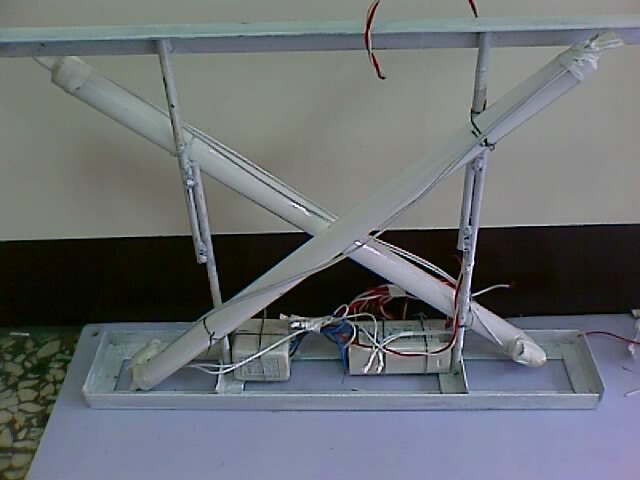The photograph shows a complex mechanical device characterized by a rectangular white frame at the bottom, with edges that extend upwards. Within this frame sit two power adapter boxes, from which multiple colored wires—specifically white, blue, and red—are entangled and partially run along two vertical metal poles situated on the right and left. These poles support another metal bracket at the top. Crisscrossing this setup are two highly reflective tubes, likely made of glass or plastic.

Additionally, the device features what appear to be four extendable arms, each paired and crossing from corners to opposite ends—one set running from bottom left to top right and the other from top left to bottom right. On the top right, a red wire prominently loops out from the power adapters, while at the bottom, a combination of red and white wires connects to a white square component. The top section of the unit has a long white bar, and the bottom section displays a white rectangle with three visible openings. Overall, the device is a sophisticated assembly of varied mechanical and electrical components.